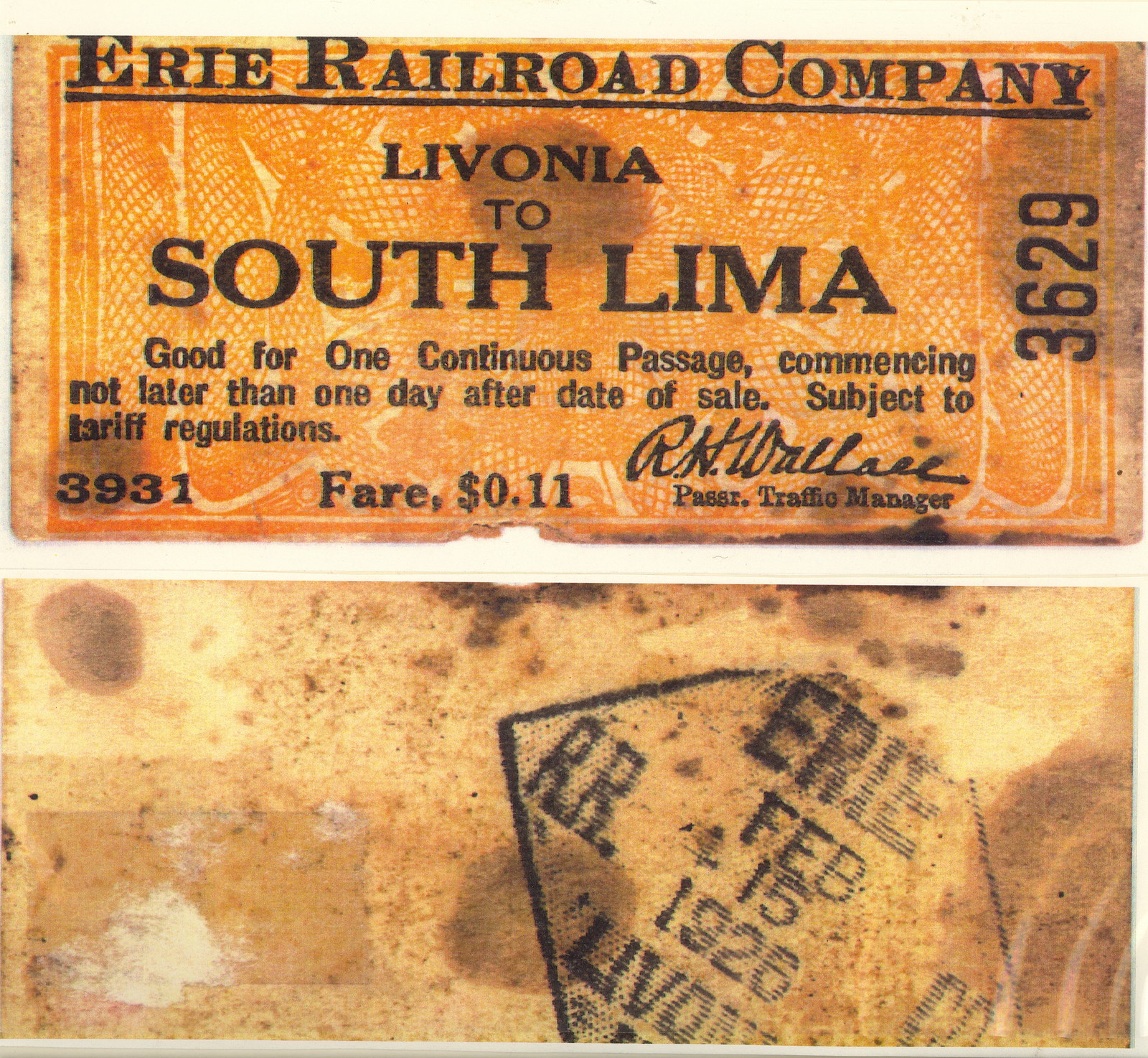The image displays a weathered train ticket from the Erie Railroad Company, presenting both its front and back. The top section of the ticket, with a faded and stained red background, features black text that reads: "Erie Railroad Company," followed by "Livonia to South Lima." It states the conditions of use, "Good for one continuous passage, commencing not later than one day after date of sale, subject to tariff regulations." At the bottom of this section, it lists the fare as "3931 fare, 11 cents" and includes a signature by a Passenger Traffic Manager, along with the number "3629" printed vertically on the right side. The bottom part of the image shows the back of the ticket, significantly worn and stained. It holds a black ink stamp within a square border that reads: "Erie, February 15th, 1926," with "RR" to the left and "Livonia" included in the stamp, indicating the ticket's usage date.